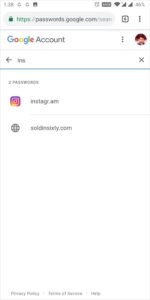The image features a predominantly white background with a blue border encompassing the entire frame. At the top, there is a search bar with a search button on the right, distinguished by a small lock icon next to it. Inside the search bar, the URL "passwords.google.com" is visible, alongside a small square icon that appears to have a plus sign inside it, followed by an ellipsis (three dots) icon, though it is somewhat blurry.

Below this, there is another box displaying "Google Account." The familiar Google logo in blue, red, yellow, and green colors is present, along with another ellipsis icon and a circular image placeholder, likely for a profile picture. Adjacent to this, there is a box with a left-pointing arrow, the number "375," and a multiplication symbol (X). 

A thicker blue line separates the sections, beneath which there are entries for two passwords. One part of the screen contains a small box featuring an image resembling a camera, colored in purple, yellow, and red, with associated text that is too blurry to read.

Further down, there's a small gray circle with a grid of squares inside it, with another indecipherable word next to it. At the bottom of the image, there appears to be text indicating "Privacy Policy" and two other small boxes, although the specifics are unclear due to blurriness.